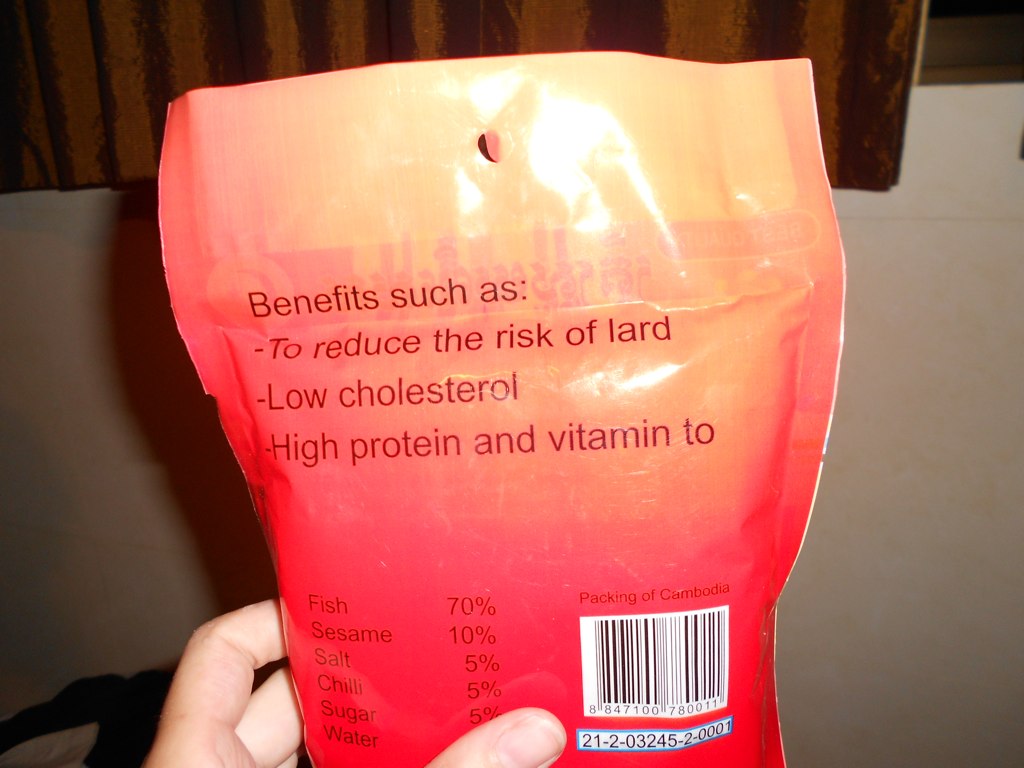This image captures a bag with a distinctive gradient design, transitioning from orange at the top to pink and red towards the bottom. The bag prominently features a UPC code located on the bottom right, with a number beneath it in a rectangle: 21-2-03245-240001. Above the bag, there is a pleated, brown curtain extending downward about an inch. The bag is resting on an off-white seat.

The text on the bag lists several benefits in bullet points: 
- Reduces the risk of "LARD" 
- Low cholesterol 
- High protein and vitamin 2 (written as "vitamin T-O")

In a smaller font, the text on the left-hand side of the bag, immediately to the right of the UPC code, reveals the bag’s contents: 
- Fish 70%
- Sesame 10%
- Salt 5%
- Chili 5%
- Sugar 5%

The word "water" is partially obscured by a person's thumb, which along with the index and middle fingers, is holding the bag.